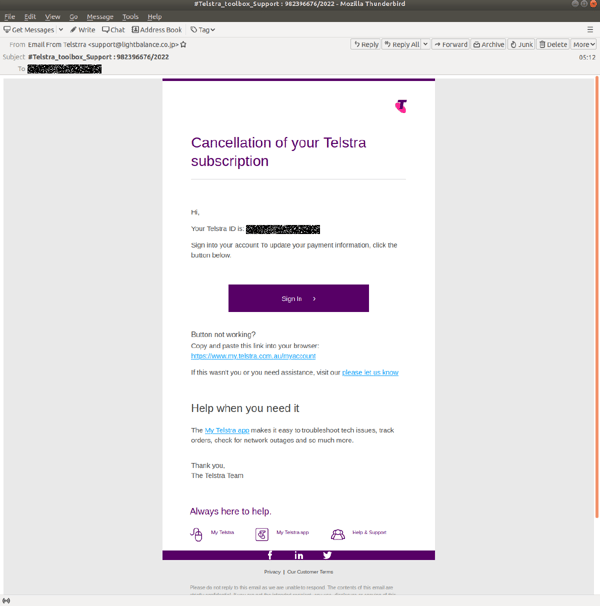The image appears to be a screenshot of an email designed to look like a web page. The page has a black header with several small, unreadable tabs. Below the header, there is a grey rectangle containing subheadings such as "address book," "chat," "write," and "get messages." Adjacent to this, on the right side, there are buttons labeled "reply," "reply all," "forward," "archive," and "delete." 

On the left, there is additional text that is too blurry to decipher, accompanied by a black box. The main content area features a grey background with a central white rectangle bordered by purple lines at the top and bottom. The title within this rectangle reads "Cancellation of your Telstra subscription."

The message body starts with "Hi," followed by a mention of an "ID" and a purple rectangle containing an unreadable number. It prompts the user to "Sign into your account to update your payment information," followed by a few illegible words. Below this, there is another purple button with unreadable text.

The message continues with a suggestion to "Copy and paste" a clickable aqua-colored address if something isn’t working. It further mentions gathering more evidence if needed but contains some indecipherable segments and a blue hyperlink.

Toward the bottom of the email, there’s a line that reads, "always here to help," followed by several small icons with accompanying descriptions that are too small to read. The footer area is purple, featuring both Facebook and Twitter icons.

Overall, the screenshot reflects an official-looking yet suspicious email, potentially a phishing attempt, urging the recipient to act upon their Telstra subscription details.